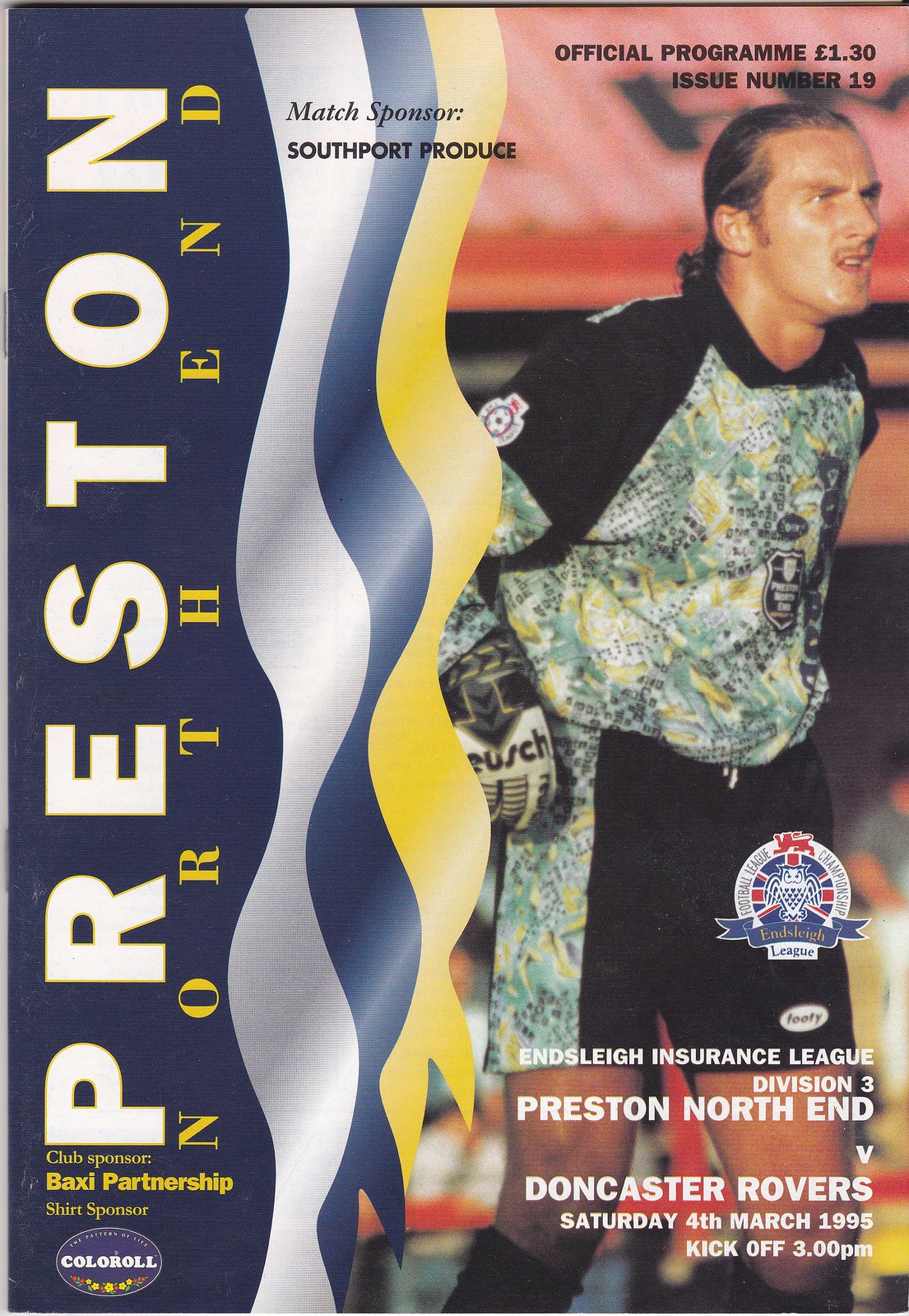This is a detailed photograph of a soccer program for a match in the Ensley Insurance League, Division III. On the left side, the program features vertical white letters spelling "P-R-E-S-T-O-N" against a blue wavy background, with "North End" written in yellow below. Further down, it lists the Club Sponsor as Baxi Partnership. Alongside, a white wavy line, blue wavy line, and yellow wavy line run from top to bottom. 

In the upper right corner, "Official Program $1.30 Issue Number 19" is prominently displayed. Below this, a photo of a white male soccer player is featured. He is donning a black uniform adorned with green, yellow, and white geometric shapes on the front and down the sides of the shorts. The player, who has short hair and black socks, is looking intently in front of him. He also wears gloves, indicating his role could be a goalkeeper.

Underneath the photo, there's a logo representing the football league championship. Below this emblem, details of the match are provided in white text: "Ensley Insurance League Division III, Preston North End versus Doncaster Rovers, Saturday, 4th March 1995, kickoff 3 p.m." In the lower left corner, "Match Sponsor: Southport Produce" and "Shirt Sponsor: Color Roll" are also mentioned.